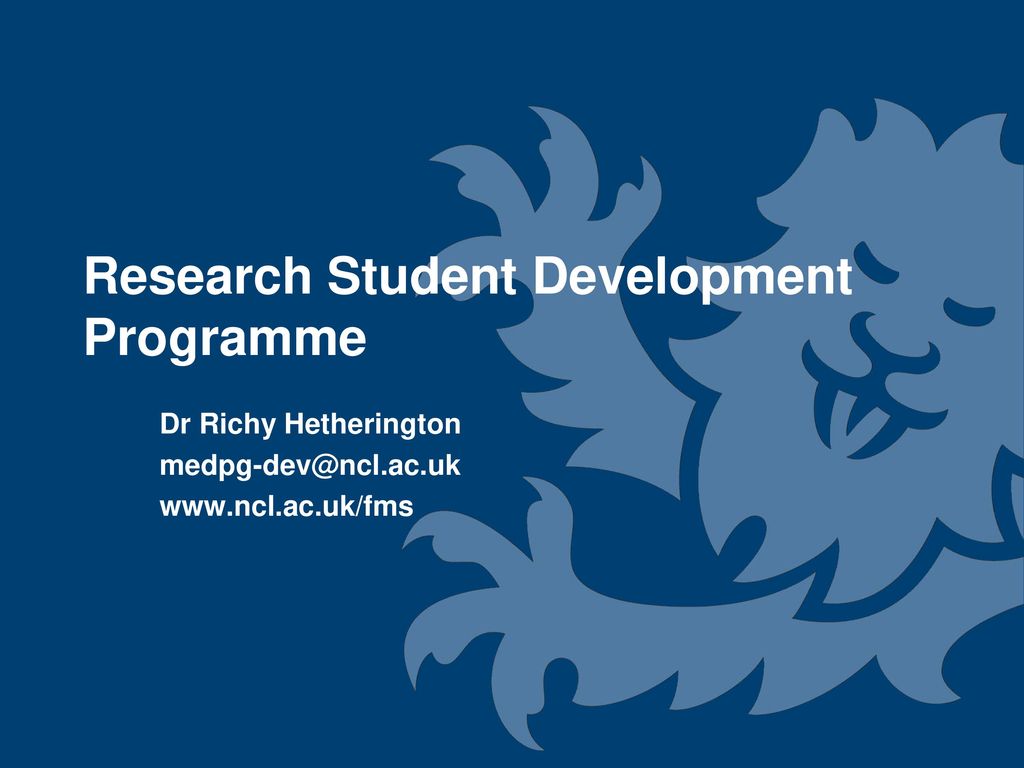This banner, possibly an advertisement, features a predominantly dark blue background with a subtly contrasting lighter blue logo that appears to be a highly stylized lion. At the center of the banner, bold white letters announce: "Research Student Development Program." Below this, also in white, it reads: "Dr. Ritchie Hetherington." Further down, the text: "MEDPG-DEV@ncl.ac.uk" is displayed, followed by the website link: "www.ncl.ac.uk/FMS." The topmost text is in a larger font size, drawing immediate attention, while the subsequent lines are presented in progressively smaller fonts.